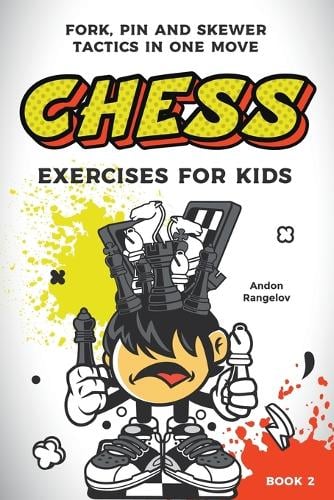This is a detailed description of a children's book with a whitish-gray background. At the top, there is a title in black letters stating, "Fork, Pin, and Skewer Tactics in One Move." Beneath this, in bold yellow letters with red shading, the word "Chess" stands out prominently. Directly below, in smaller black lettering, it reads, "Exercises for Kids."

The central illustration features a cartoon drawing of a boy who appears to be composed solely of his head, arms, legs, and feet. He is holding two chess pieces, one white and one black, in his hands. The boy is wearing untied gym shoes and is depicted standing on a chessboard. His tongue, which is red, is playfully sticking out. He has long, black hair, and resting atop his head is a partially open chessboard from which both white and black chess pieces are emerging.

In the bottom right corner, there is a red section of the cover that indicates, "Book Two."